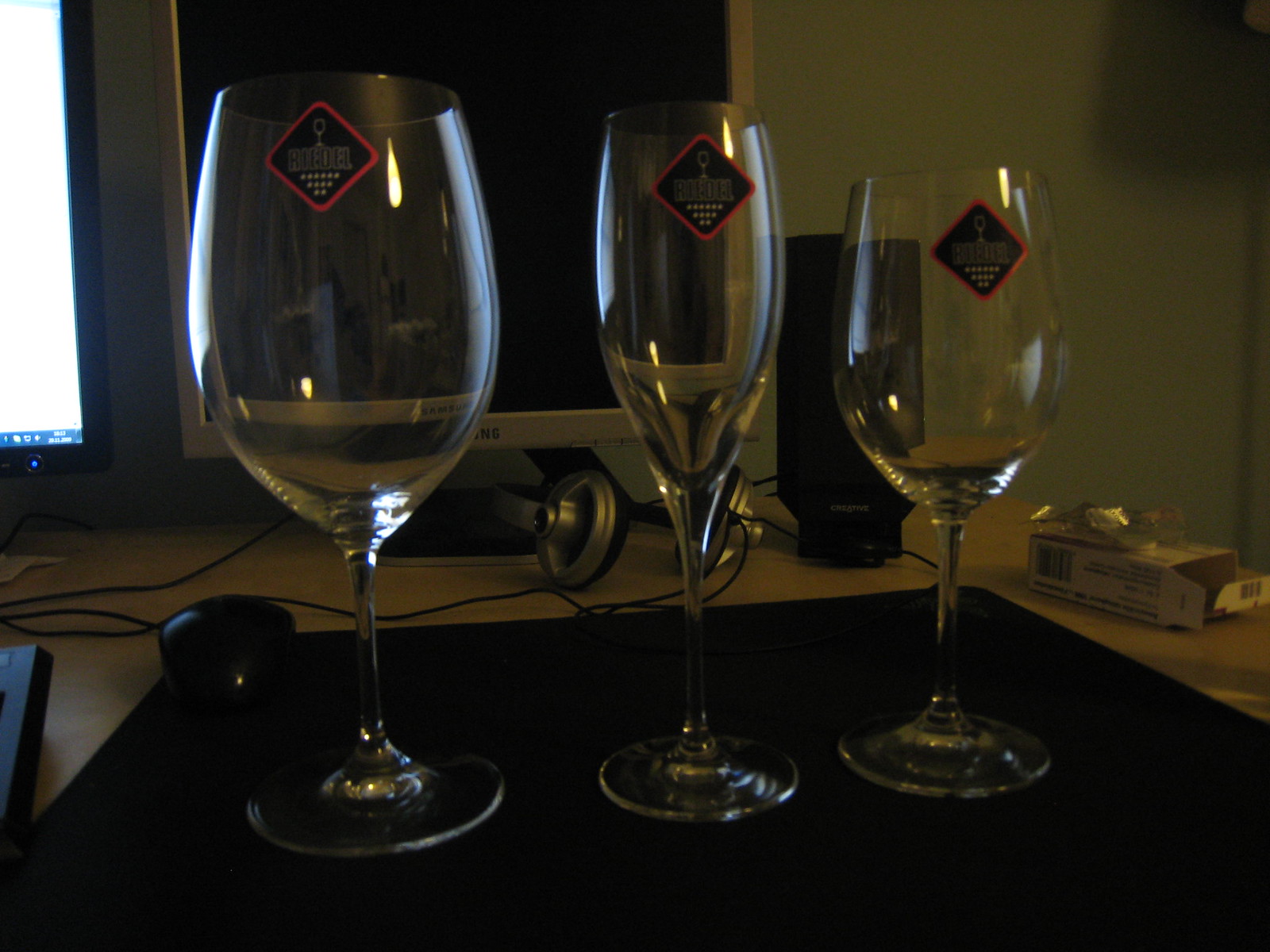This photograph showcases a detailed setup on a computer desk, featuring three distinctive wine glasses of varying sizes, all adorned with a black, white, and red logo in the shape of a yield sign. These glasses are neatly positioned on a black mouse pad situated in the center of the image. Starting from the left, we observe a broader, taller wine glass, followed by a slender, tall wine glass, and finally, a shorter but wider one. Behind these glasses, slightly off the mouse pad, lies a pair of gray headphones with a microphone. The background includes several electronic components: a partial computer screen to the left, an old white-framed monitor, and a speaker. Adjacent to the mouse pad on the right, there appears to be an opened package, possibly a medicine blister pack. The desk itself is a tan color, contrasting with the black mat. The overall setting is clearly indoors, with a gray wall forming the backdrop.